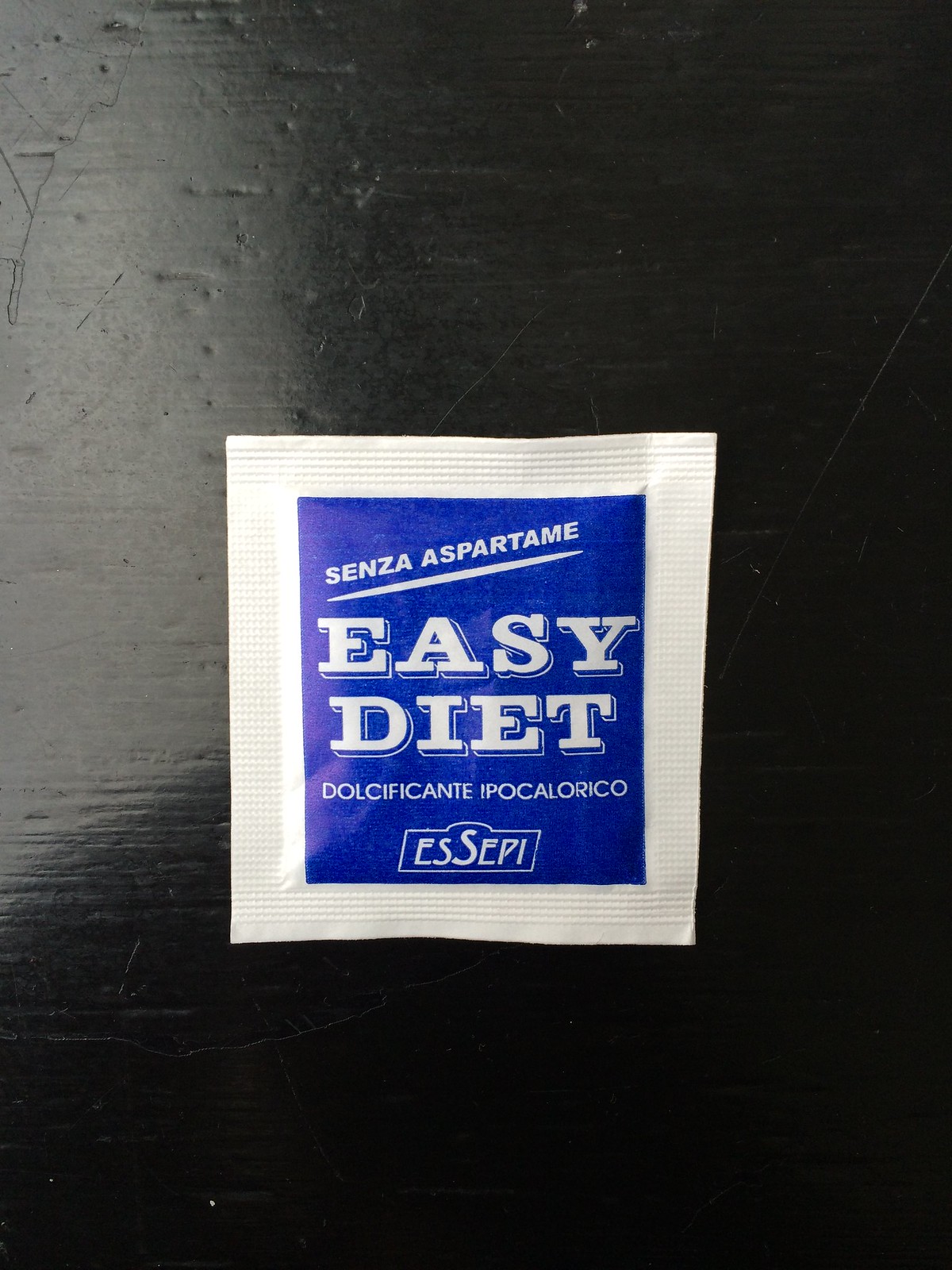This digital photograph, captured in portrait orientation, showcases a singular, detailed view of a white packet positioned on a black wooden table with visible light reflections in the upper left-hand corner. The black table, with chips and indentations painted over, forms a stark contrast against the packet, emphasizing its features. At the center of the image is the packet, featuring a prominent square blue section with various inscriptions. The top of the blue square is slightly angled and reads "Senza Aspartame," beneath which is written "EASY DIET" in capitalized, bubble-like letters. Further below, the phrase "DOLCIFICANTE IPOCALORICO" is displayed. The packet, designed for easy ripping, has ridges stamped along its edges and a logo at the bottom that reads “ESSEPI,” with the second “S” notably larger, set within a rectangular frame with a domed top. The overall appearance suggests that this packet is a low-calorie sweetener.